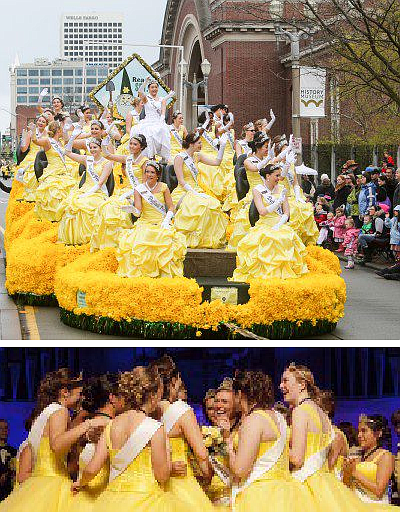In this vibrant parade scene, a float adorned with bright yellow flowers, possibly buttercups, makes its way down a bustling street. The parade spectators line the sidewalks, eagerly watching as a group of women dressed in banana-yellow gowns with ruffles and white gloves pass by. Each woman wears a sash, possibly representing different counties or states, and a tiara. The float features a majestic centerpiece—a young lady elevated above the rest, wearing a white gown, sash, and tiara, signifying her as the queen. Various signage can be seen around the float, including an image of a gnome with a shovel. The women, whose hair colors range from blonde and brunette to redhead, wave gracefully to the crowd, their smiles capturing the festive spirit of the event. The backdrop includes a charming mix of buildings, adding to the parade’s lively atmosphere. Overall, this beautifully captured moment showcases the elegance and joy of the parade participants and the spectators' delight.